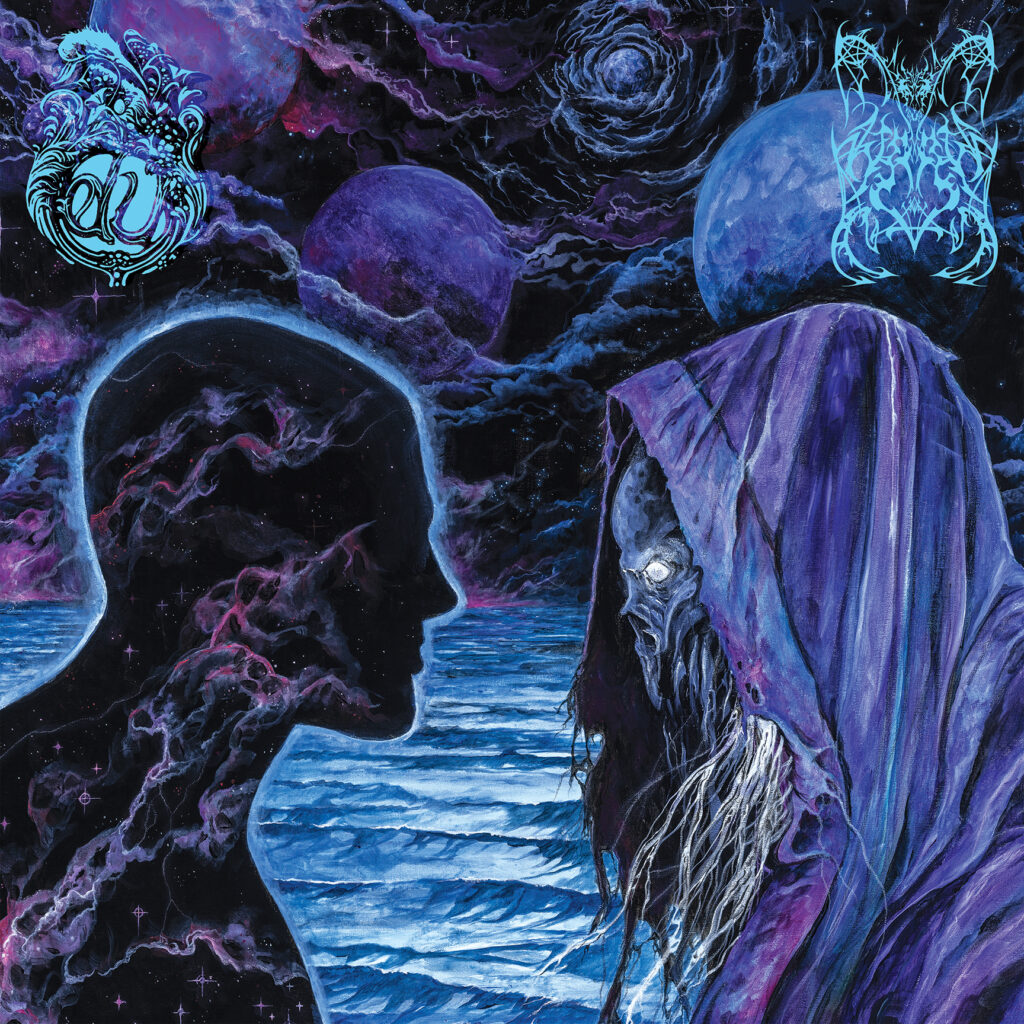This square painting vividly captures a haunting scene. On the right, a grotesque, skeletal figure looms with a hollowed face, its white, stringy hair cascading from beneath a hooded cloak rendered in deep blues and purples. The creature’s glaring white eyes are fixed on a black silhouette of a human figure on the left. This human figure, depicted from the chest up, is entirely filled with intricate swirls that mimic a night sky, complete with stars and cosmic clouds in purples, reds, and blues. The background is dichotomous, with the bottom half depicting tumultuous blue water, while the top half portrays a stormy night sky filled with dark clouds and multiple purple-blue moons. Above both figures are ornate, light blue emblems: on the left, a rounded, frilled logo bearing the initials “EK,” and on the right, a delicate, butterfly-like line drawing. This evocative composition, drenched in eerie and creeping tones, immerses the viewer in a disquieting atmosphere of otherworldly dread.